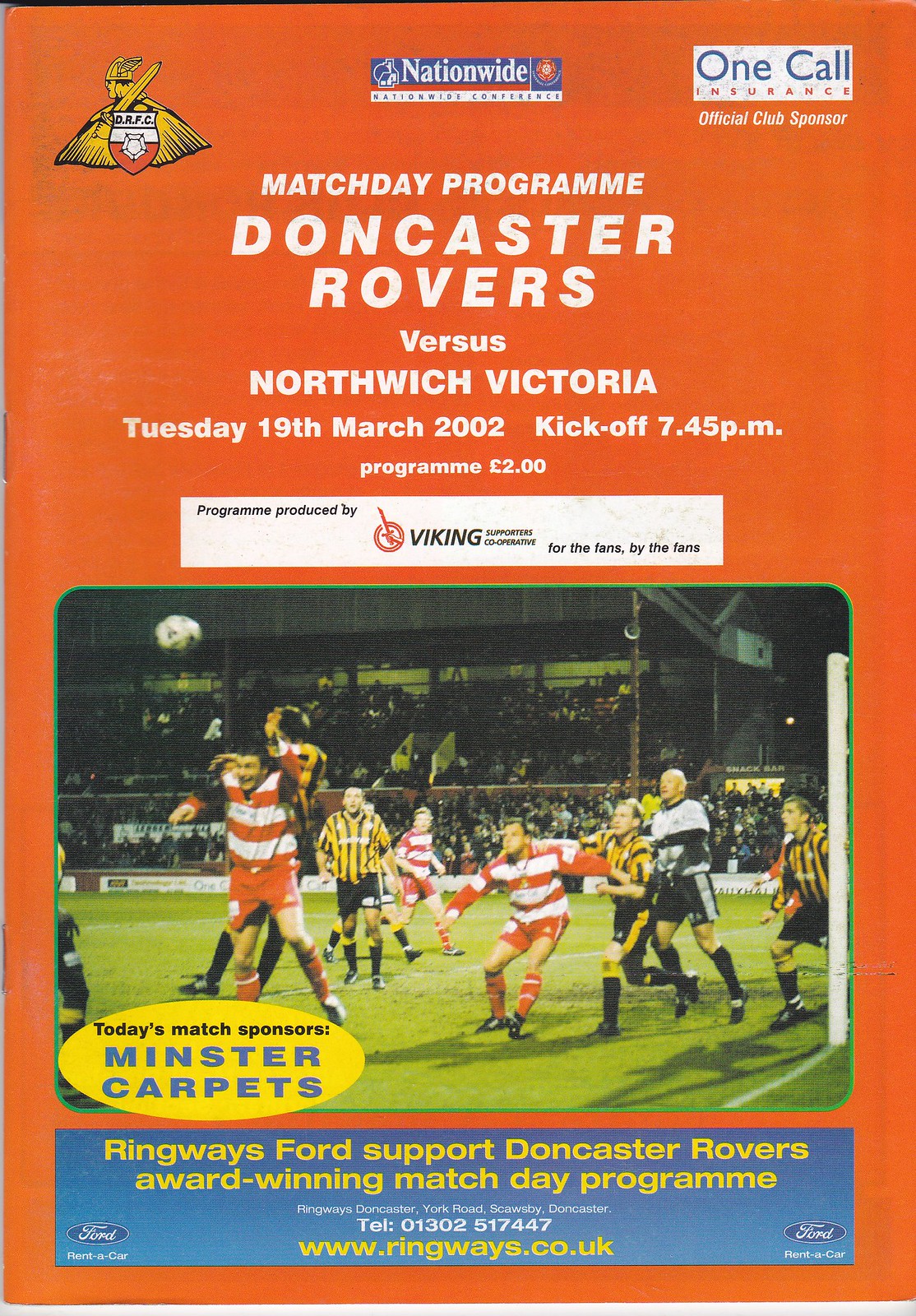This image is an advertisement for a soccer game, set against an orange background. It prominently features a variety of sponsor emblems and ads. In the upper portion, a yellow, red, and white emblem sits in the upper left-hand corner, though it's difficult to identify. Centrally placed is the "Nationwide" title in white over a blue background. On the right, the text "One Call Insurance" appears in red and blue against a white backdrop, with the phrase "Official Club Sponsor" underneath.

Across the top center, the caption reads in bold white text: "Match Day Program, Doncaster Rovers versus Northwich Victoria, Tuesday, 19th March 2002, kickoff 7.45 p.m., program two pounds (or two euros depending on the source)." Below this, it clarifies, "program produced by Viking." 

The main body of the image highlights an action-packed soccer scene. Players from Doncaster Rovers, identifiable by their red and white striped jerseys, and Northwich Victoria in yellow and black striped jerseys, are captured mid-play with the soccer ball blurred due to motion. 

A standout yellow oval overlay near the center states, "Today's match sponsors Minster Carpets." Towards the lower section, a blue background contains the text, "Ringways Ford supports Doncaster Rovers award-winning Match Day Program," along with the contact number 01302 517447 and the website www.ringways.co.uk. 

The colors prevalent in this image include black, white, red, orange, gold, yellow, green, gray, and blue, creating a vibrant and dynamic promotion for the match.